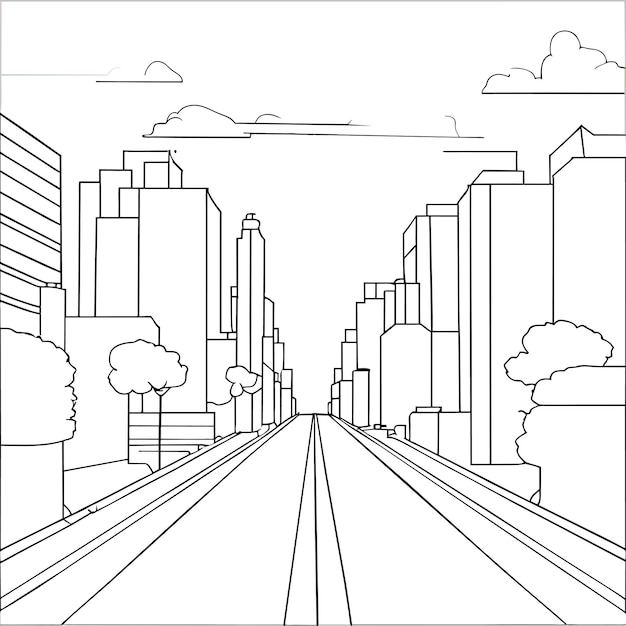The image appears to be an intricate black-and-white illustration resembling an uncolored page from a coloring book. It features a perspective drawing of a cityscape with tall buildings flanking a two-lane road that stretches into the distance, converging slightly below the center of the image. The buildings are depicted as flat rectangles with minimal dimension, contributing to a clean and geometric aesthetic. Along the roadway, there are a few trees and possibly some bushes, providing a touch of nature amidst the urban scene. Simplified clouds float in the sky above. Every element in the image, from the buildings to the trees and clouds, is rendered with consistent line weight, devoid of shading or intricate details, emphasizing the sketch-like quality. The overall composition is exact and orderly, reminiscent of something one might print out for children to color in school.